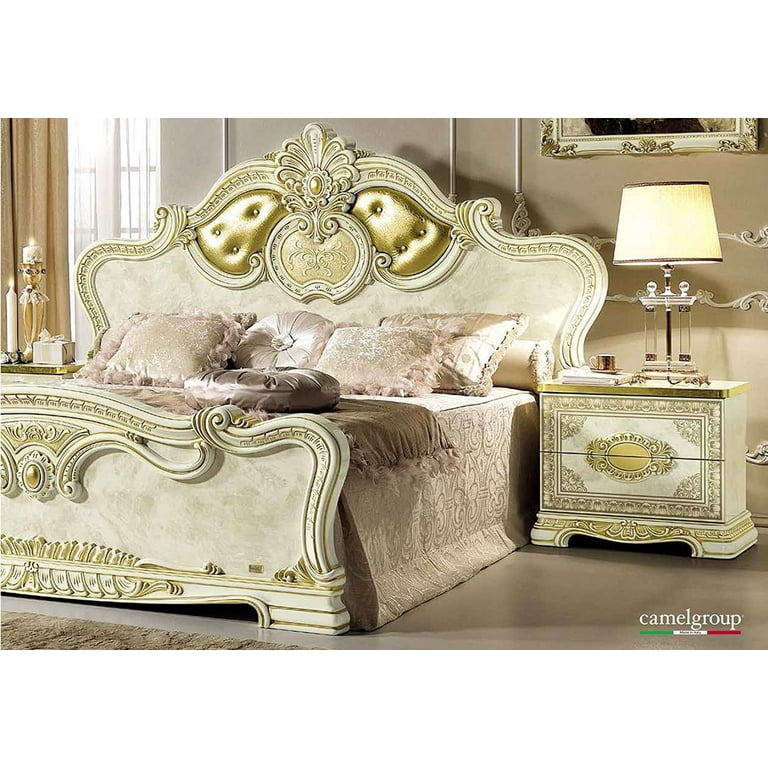This image depicts a lavish and ornate Italian-style bedroom, exuding a rich Baroque or Gaudi influence. At the center is a king-size bed, characterized by an elaborate wooden frame with a gold-cushioned headboard. The bed is draped in soft, plush bedding, including pinkish covers and a selection of throw pillows, notably two circular ones. On either side of the bed are matching bedside tables, designed with intricate, stylized Italian patterns and adorned with floral gold-etched details against a central white backdrop. The right nightstand features a lamp and a small teacup or coffee cup, while the left nightstand is decorated with lit, fancy candles. Behind the bed, the beige wall holds a framed picture, contributing to the room's overall gaudy, yet sumptuous decor.